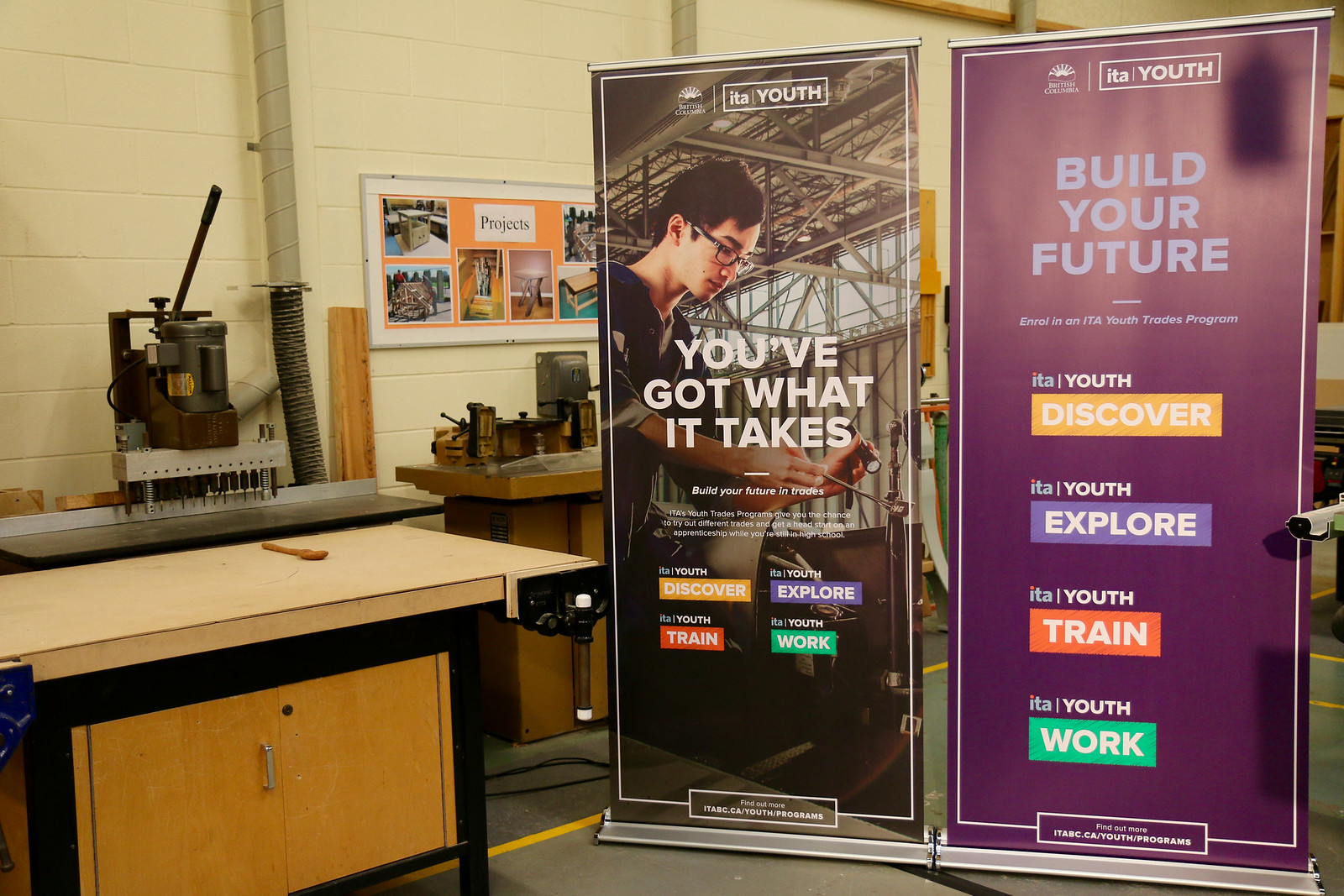This photo is a detailed view of a job fair display set in what appears to be a workshop or classroom. On the left side, there's a workbench equipped with machinery, including a vise and a drill press, along with a lever tool situated on the counter. The workbench also features cabinet doors below, with the left door having a vertical silver handle and the right door equipped with a lockable keyhole. 

Central to the image, a bulletin board labeled "Projects" decorates the wall, showcasing various images of completed woodworking projects and tables. Beneath this bulletin board, another work table supports additional vices and levers. 

Dominating the right side of the photo are two tall, pull-up banners promoting the ETA Youth trades program. The first banner, on the left, depicts an Asian male wearing safety goggles. He is engaging in a hands-on activity involving a pipe, using a flashlight and a tool. The banner prominently displays the slogan "YOU'VE GOT WHAT IT TAKES" in all caps, followed by smaller, less legible print, and a series of colored rectangles—yellow, red, purple, and green—each inscribed with the words Discover, Train, Explore, and Work, respectively. Each rectangle is accompanied by the ETA Youth logo.

The second banner, on the right, features a dark blue background with the message "BUILD YOUR FUTURE" written in light blue, all caps. Below, it includes a call to action to "email us at ETA Youth trades program" and mirrors the first banner's colored rectangles and corresponding words: Discover, Explore, Train, and Work, again each tagged with the ETA Youth logo.

The overall scene is set against a white cement wall, reinforcing the industrial and educational environment of the workshop.